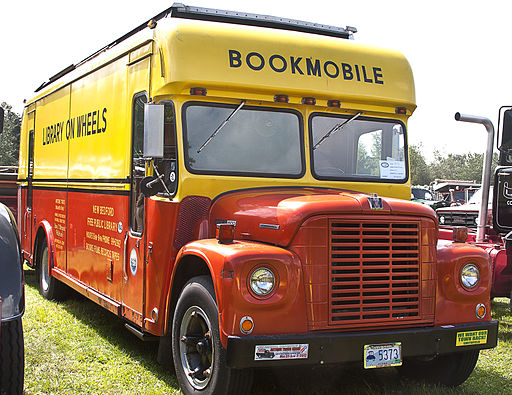This photograph captures a detailed and lively scene of a vintage bookmobile, parked on a lush, green grassy field under a clear white sky. The vehicle stands prominently at the center, characterized by its vivid red lower half and bright yellow upper half, reminiscent of a school bus yet styled like an old fire engine. Above the driver's windows, a sign board reads "Bookmobile," and on the side, it proudly bears the title "Library on Wheels," indicating its purpose as a mobile library. The bus, which features black tires, windshields, side view mirrors, and headlights, also carries a license plate numbered 5373. Additional bumper stickers flank the plate. Surrounding the bookmobile are various other vehicles, including buses, trucks, and minivans, with trees dotting the background and casting shadows along with sun rays illuminating the scene. This picturesque setting, possibly a field or an open ground, suggests that the bookmobile might be displayed as a nostalgic exhibit rather than in active service.